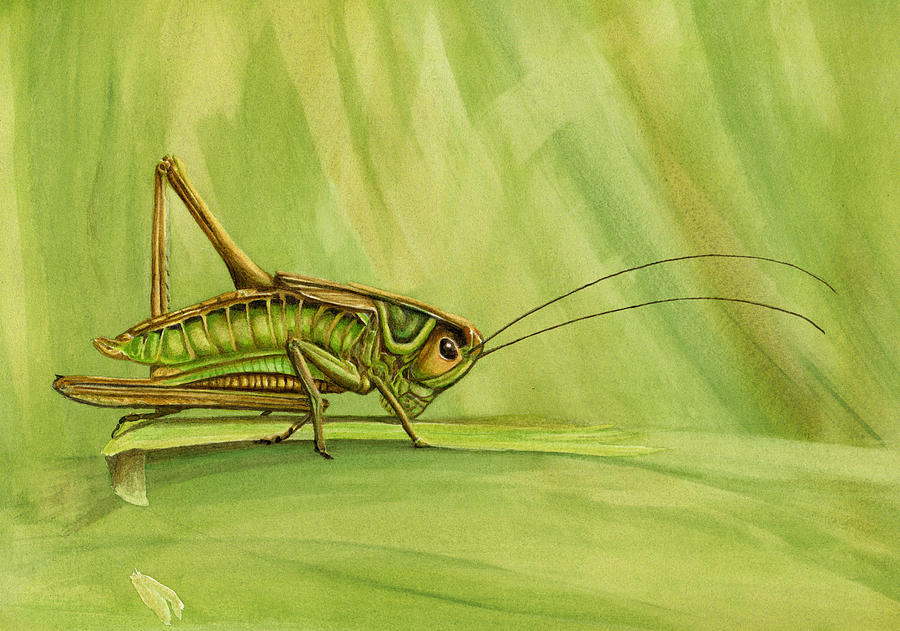The artwork depicts a vividly detailed grasshopper set against a richly textured green background. The background features an array of green hues, including lime, dark, olive, and yellow green, all interspersed with white streaks, creating a dynamic, stripe-like pattern that covers the entire canvas. The grasshopper is perched on a singular, thin leaf, positioned slightly left of center. From a side-view perspective, the grasshopper's body faces right, revealing its intricate form. It has black eyes and long, slender black antennas. The creature's body and legs showcase a blend of greens and yellows, with certain parts of the legs displaying a transition from greenish to yellowish tones. Some of its legs are positioned on its back, while others are tucked beneath, and its front legs seem to clasp the leaf, creating a sense of lifelike readiness. The detailed rendering of the grasshopper, likely created with colored pencils, is a testament to the artist's meticulous attention to detail, capturing the essence of the insect's natural habitat among the greens.